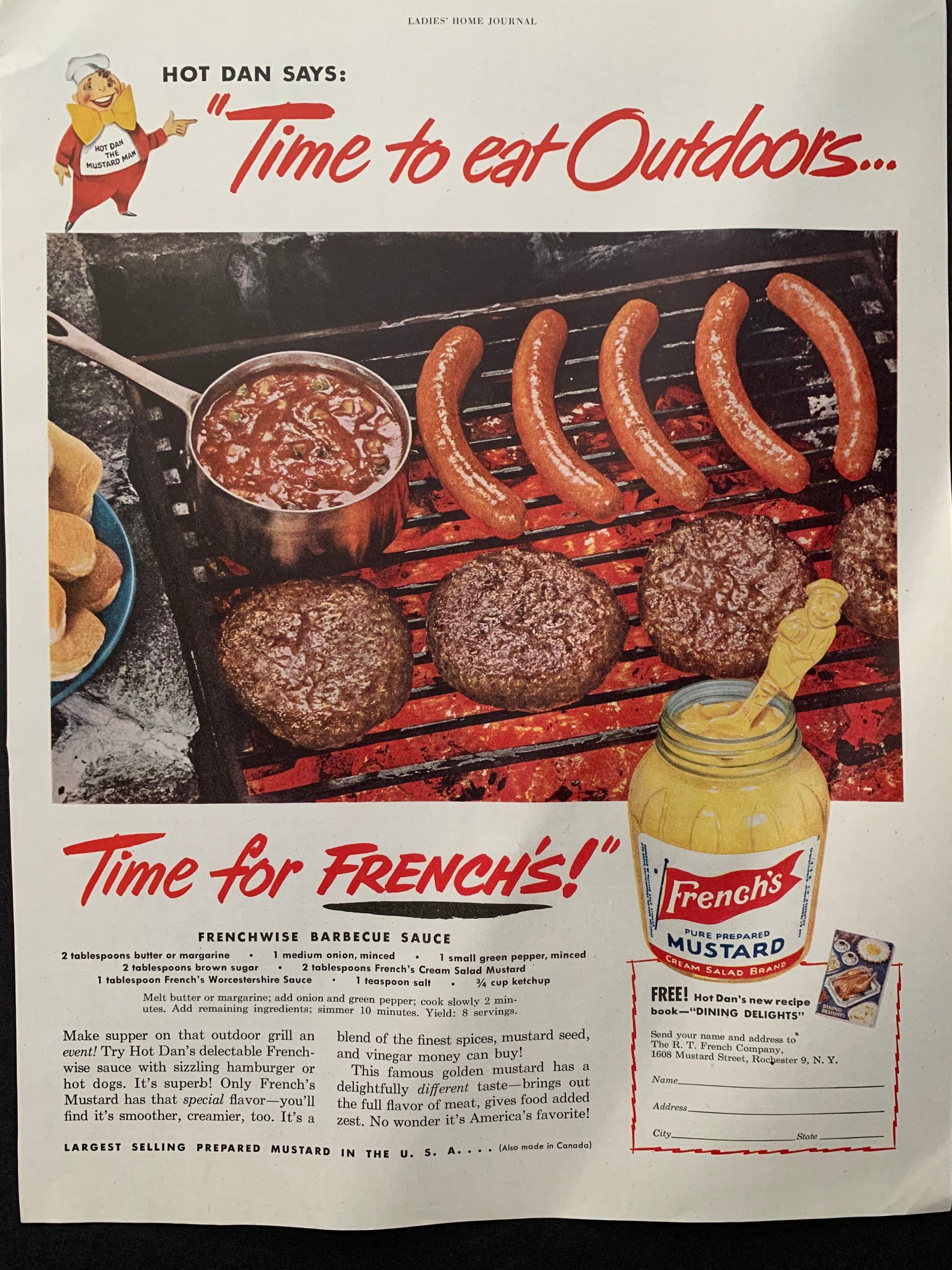The poster predominantly features white with a black border at the bottom. The top of the poster reads "Ladies Home Journal," while on the top left, there is a vibrant illustration of a cheerful mascot named Hot Dan. He is depicted wearing a white hat, a red outfit, and a large yellow bow tie, smiling and pointing to the right, with the text beside him saying, "Hot Dan says, Time to eat outdoors."

Below the mascot, there is a tempting image of an outdoor barbecue scene featuring a black grill loaded with food. The grill is cooking four brown beef patties and five grilled hot dogs, along with a silver pot containing a red sauce or stew. Adding more detail, the grill also has hot dog buns and a jar of French's mustard present, indicating it is an advertisement for French's mustard. The mustard jar, labeled "French's Pure Prepared Mustard," is prominently open, and the French's logo is displayed as a giant red flag with text across it.

Below the grilling scene, another red banner reads, "Time for French's," along with a recipe for French-wise barbecue sauce, listing the ingredients and preparation steps. The overall color palette of the poster includes red, brown, yellow, pink, white, and black, creating an inviting and appetizing appeal. This full-page ad, likely from a magazine or as an outdoor poster, compellingly promotes the joy of outdoor dining with French's mustard.